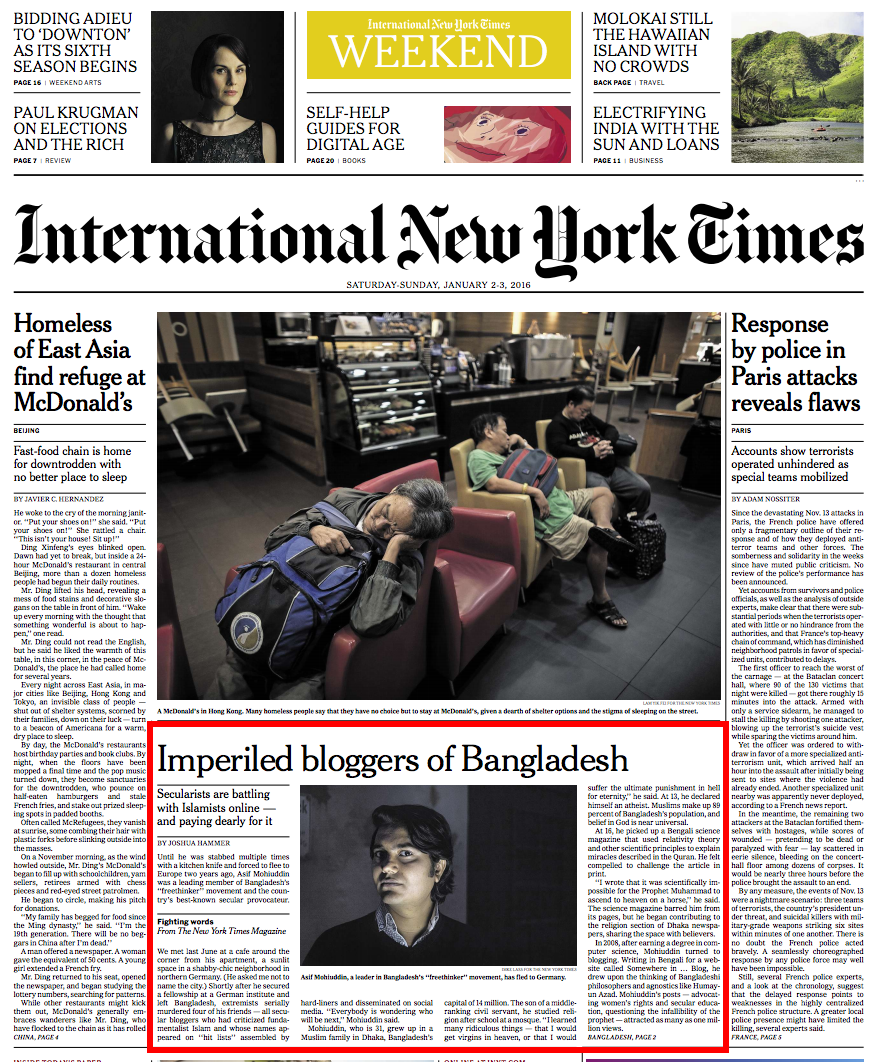Front page of the International New York Times Weekend Edition for January 2nd-3rd:

At the top of the front page are two notable columns. The first bids adieu to the TV series "Downton Abbey," while the second features Paul Krugman discussing elections and economic disparities. The title “International New York Times Weekend Edition” is prominently displayed in white text on a yellow background. Beneath this, there's a headline about a "Self-help Guide for the Digital Age."

To the right, there are two smaller features. One highlights "The Malachi: The White Island with No Crowds" on the back page of the travel section. The other discusses "Electrifying India with Solar Loans."

Below this, the newspaper’s name is written in an elegant script, with the edition date in small text. A line runs horizontally across the width of the paper.

On the left side of the front page:

- An article titled "Homeless of East Asia Find Refuge at McDonald's." The piece is accompanied by a sizeable image depicting a group of Asian people inside a McDonald's. The setting resembles a Starbucks, with patrons sitting comfortably, their backpacks over their laps.

Below this:

- An article titled "Imperiled Bloggers of Bangladesh," outlined with a red border. The piece highlights how secularists are at odds with Islamists and paying dearly for their outspokenness.

On the right side of the front page:

- An article titled "Response by Police in Paris Attacks Reveals Flaws." It details how terrorists operated unhindered even as special teams were mobilized.